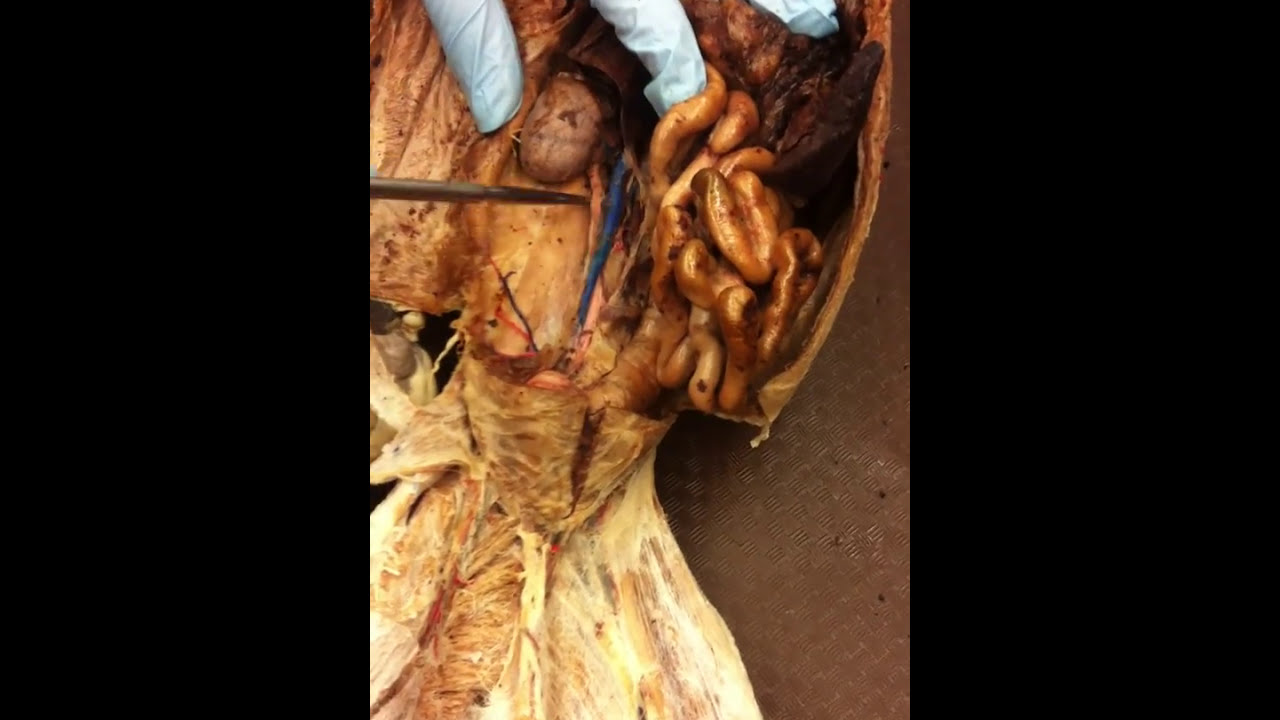The image is a color photograph in portrait orientation, centrally inset into a black landscape-oriented background. It depicts a detailed scene of a dissection, rendering the head of either a person or an animal in a representational realism style. The focal point near the top of the photo showcases a blue-gloved hand with three fingers visible, examining a central round object—described by one as resembling a walnut—using a silver tool directed from the left. The dissection reveals intricate anatomical structures: gray matter, likely brain tissue, lies within the skull, beneath which extends a neck-like structure exhibiting ligaments and skin. The background features a brown hue, compounding the intriguing and somewhat ambiguous nature of the examined tissue, which could be either biological remains or botanical growth.